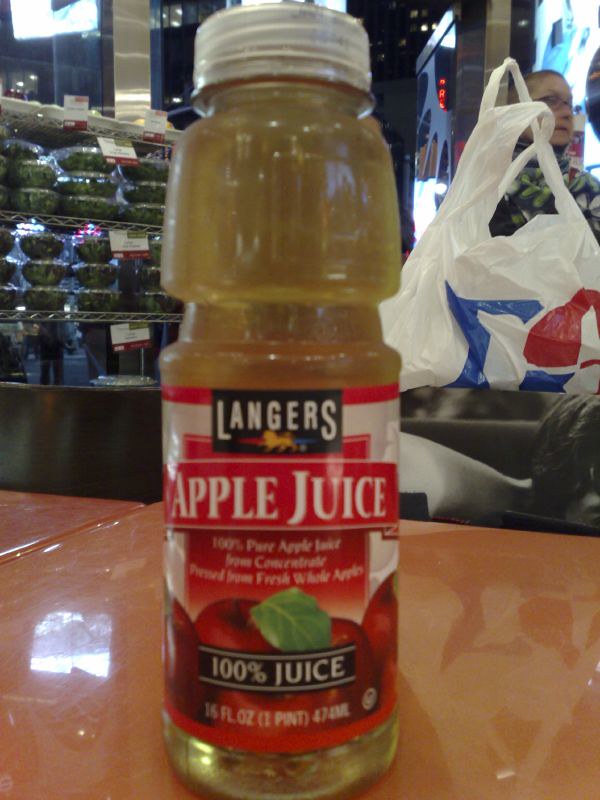In this image taken inside a deli or small grocery store, a bottle of Langer's 100% apple juice, 16 fl oz (one pint), is prominently placed on a shiny, tan-colored table in the center. To the left, there are two shelves holding stacks of clear salad bowls, each with multiple layers of salad; nine bowls are visible, arranged in stacks of three per shelf. Above these shelves, a mirror or very reflective surface enhances the scene. To the right of the apple juice, a white plastic bag with blue and red markings rests slightly higher in the frame. The face of a person with glasses, possibly a woman with close-cropped hair, appears in the upper right corner, illuminated by light from behind her head. She seems to be engaged in a conversation with someone not visible in the image.